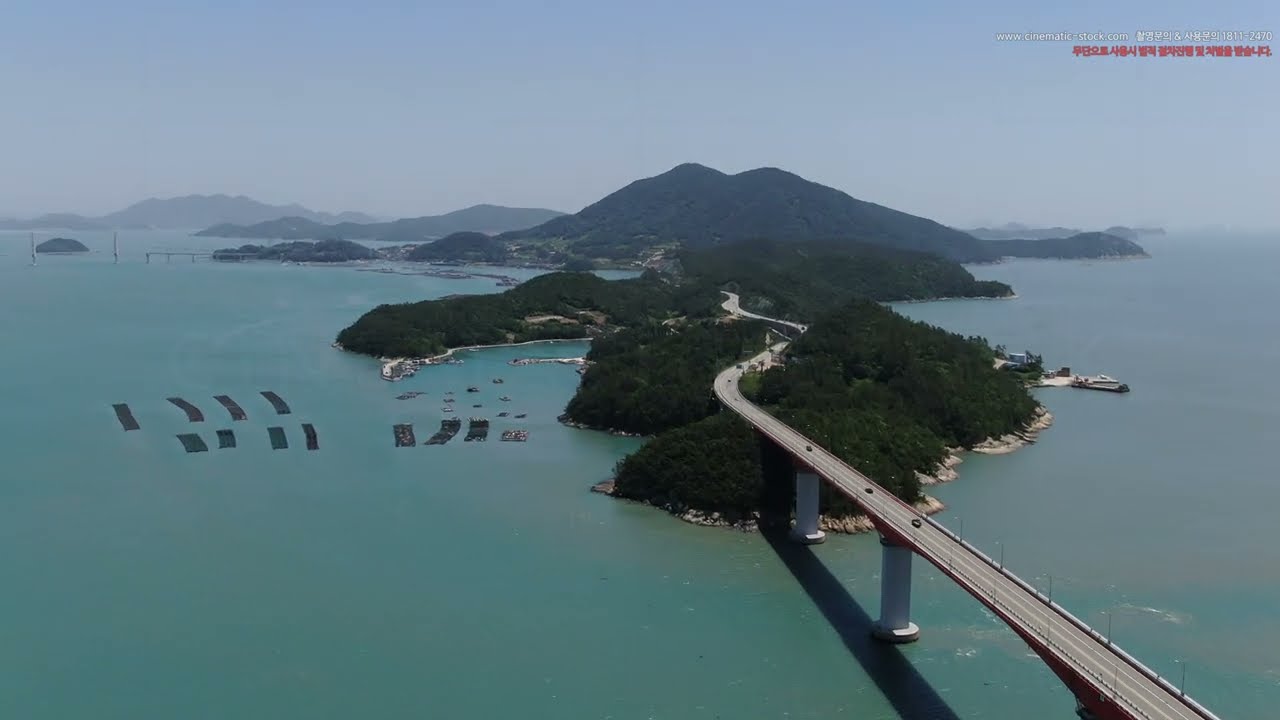The image is a detailed, color landscape photograph captured from an aerial perspective, likely using a drone. Central to the composition is a narrow bridge with three supporting pillars, extending over a body of clear aqua blue water that exhibits hints of green. The bridge leads into a lush, tree-filled island, which is dominated by a two-peaked mountain in the background. Further along the horizon, additional smaller mountains can be seen. Surrounding the island are several patchy, rectangular, and black objects on the water's surface that seem to function as moorings for boats. To the left of the island, small boats can be observed along with a dock that hugs the mountainous terrain. Overhead, the sky is a blue haze, mingled with clouds and a faint fog, giving the scene a dreamlike quality. The top right corner of the image features a URL and some text in Mandarin, suggestive of a promotional context for an engineering project. The overall style of the photograph leans towards representational realism, capturing the serene yet intricate details of the landscape below.